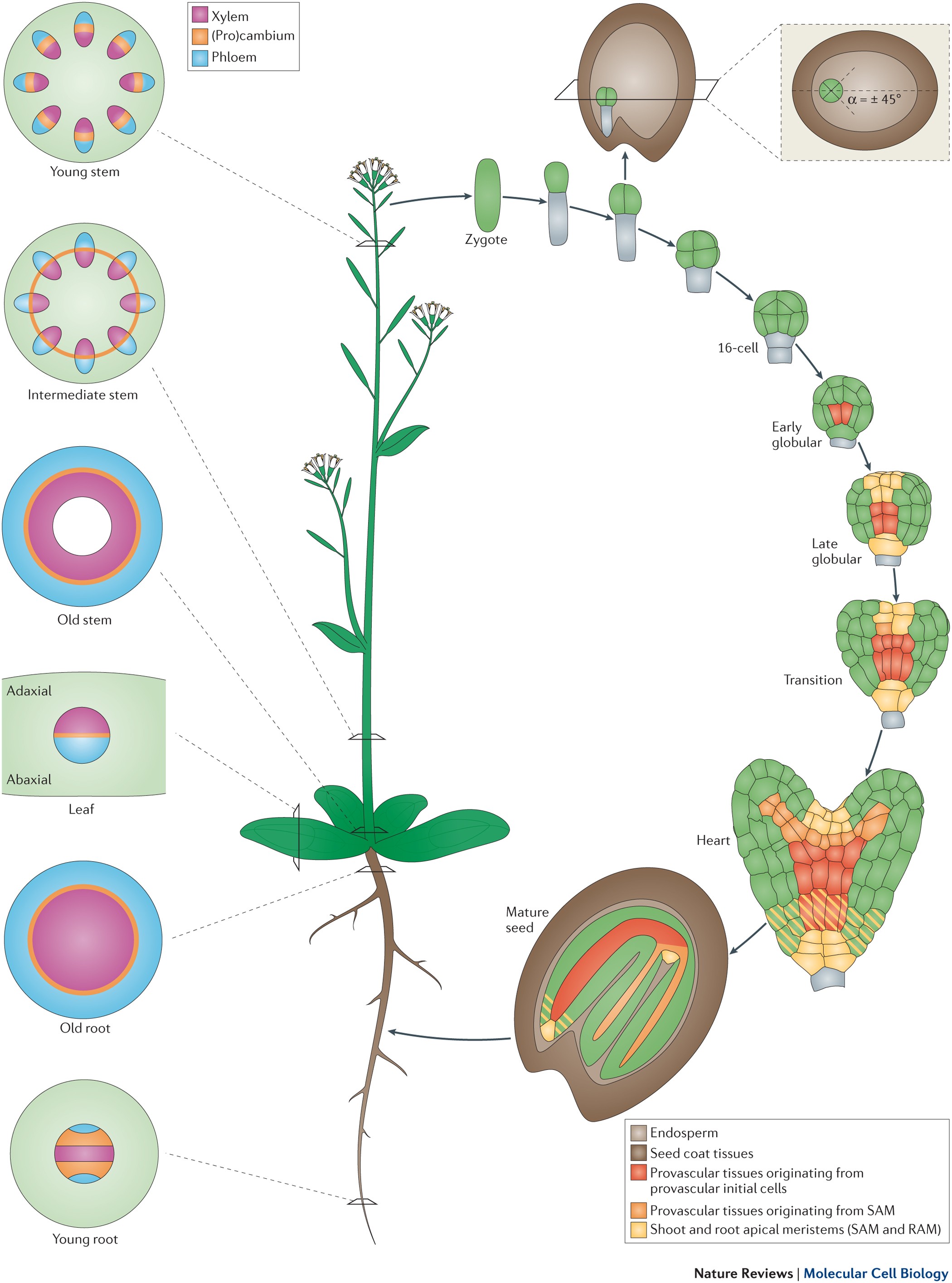This image features a detailed, cartoonish diagram against a white background, illustrating the life cycle and anatomy of a flowering plant. At the center stands a relatively tall plant with sporadic leaves and three sections bearing small white flowers. The depiction includes a prominent long root system with short branches extending from it.

Encircling the plant, there is a visually engaging representation of the plant's growth stages in a circular sequence, meticulously labeled from early to late development. This progression showcases the zygote at the flower's top, which duplicates into 16 cells, evolves into early and late globular stages, transitions into the heart stage, then matures into a seed, completing the cycle back at the root. Detailed annotations such as "young stem," "intermediate stem," "old stem," "adaxial leaf," "abaxial leaf," "young root," and "old root" highlight different plant parts and their stages of growth.

Additionally, on the left side of the image, there are smaller circular diagrams pointing to various components of the plant, providing in-depth information about each part. These annotations include terms like endosperm, seed coat tissues, probascular tissues originating from different initial cells, and references to the shoot and root apical meristems (SAM and RAM).

Overall, this diagram, titled "Nature Reviews Molecular Cell Biology," serves as an educational tool, detailing the intricate stages of plant growth, from seed germination to maturity, and the various anatomical parts involved throughout the plant's lifecycle.